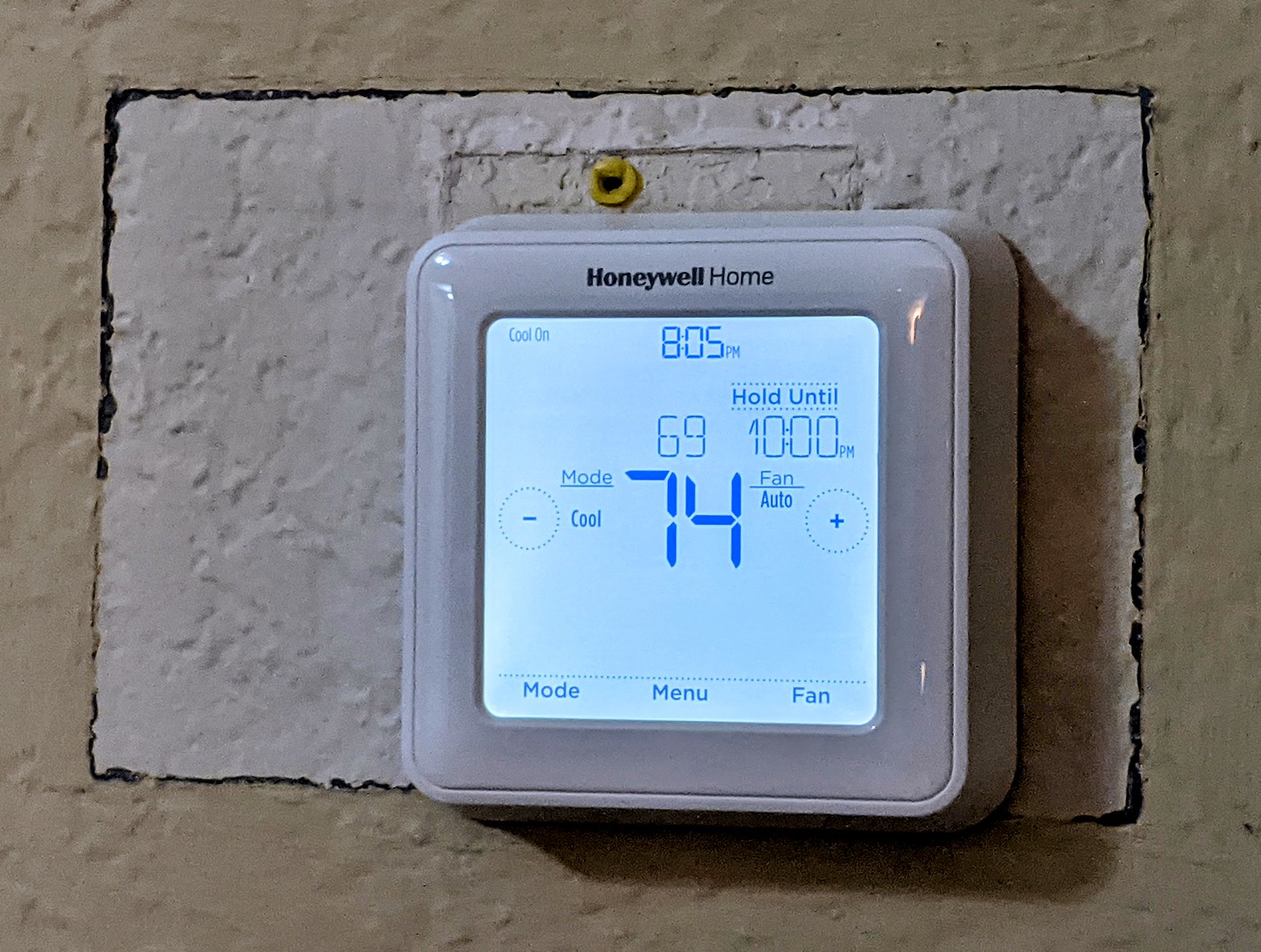A dark gray concrete wall serves as the backdrop for this scene. Centrally affixed to the wall is a lighter gray slab, secured with a gold-colored screw. Mounted on this slab is a sleek, light gray thermostat bearing the brand name "Honeywell Home" in black lettering. The thermostat features a glass front and displays a user interface with a light blue background. 

On the screen, the words "Cool On" appear in blue letters at the top, accompanied by the current time, 8:05 PM. Additionally, the thermostat indicates a temperature setting of 69 degrees Fahrenheit with a hold status until 10:00 PM. Below this, there is a small dotted circle with a minus sign, adjacent to the word "Mode" followed by a linear separator and the word "Cool." A larger, more prominent number "74" is displayed, indicating the current room temperature. The screen also shows the status of the fan as "Auto" next to another line and a plus sign.

At the bottom of the display, a dotted line separates options for "Mode," "Menu," and "Fan," all presented in blue letters within the compact, sophisticated thermostat box.